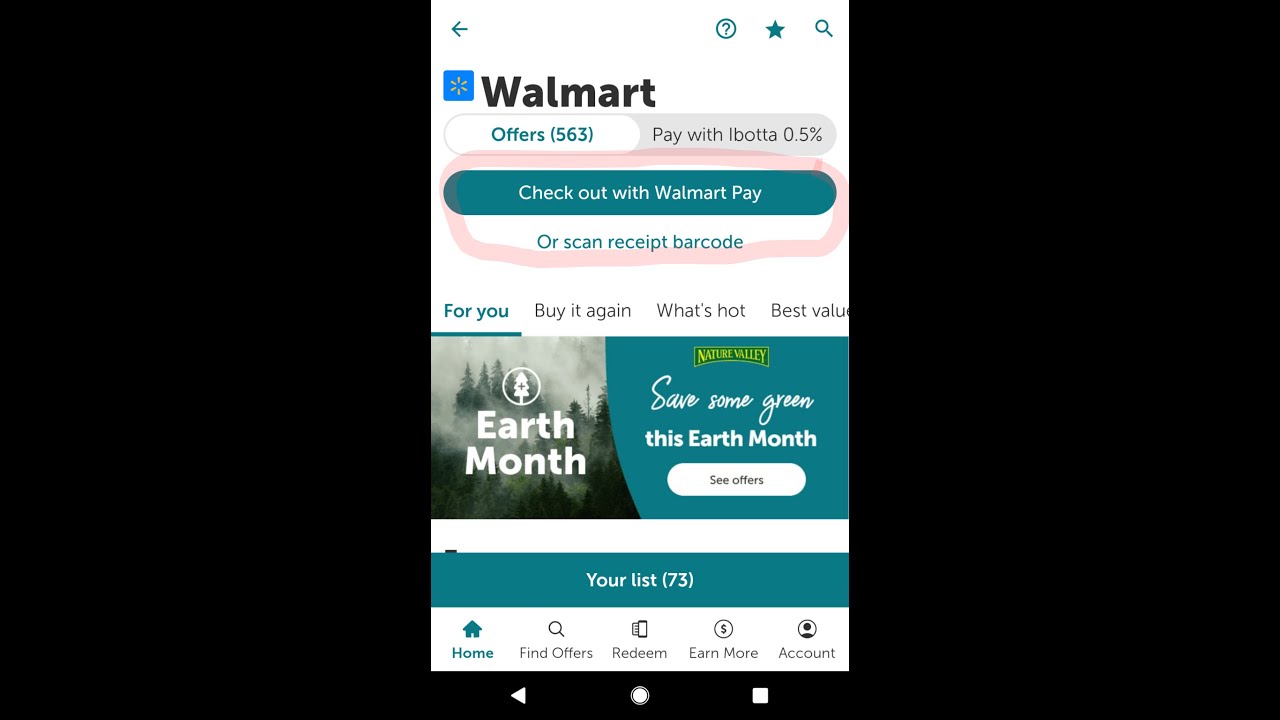A meticulously edited photo centers around a large black square backdrop, occupying most of the frame. Positioned precisely in the middle of this black space, a mobile screenshot of the Walmart app stands out. The stark contrast is emphasized by the extensive empty black spaces flanking the screenshot on both the left and right sides. At the bottom edge of the app screen, the familiar black phone navigation bar is visible, featuring a left-pointing arrow for back navigation, a central circle, and a square icon on the right.

The Walmart app interface displayed has a pristine white background. Dominating the top left corner is the iconic Walmart logo, accompanied by the name "Walmart" in prominent, bold black letters. Directly beneath this header are two distinct buttons: "Offers 563" on the left and "Pay with Ibotta 0.5%" on the right. Below this section, an eye-catching, large blue bar prominently reads "Check out with Walmart Pay." Adding a focal point, a red circle has been edited into the image to highlight and draw attention to the "Check out with Walmart Pay" button. The overall composition emphasizes the key features of the Walmart app in a clear and visually engaging manner.